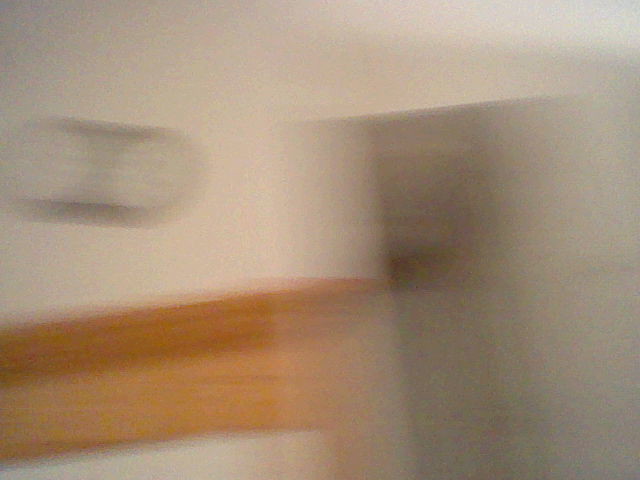The image portrays a very blurry scene, making details hard to discern. In the bottom left corner, there appears to be an L-shaped structure made of light wood-toned material, possibly serving as a door frame. Adjacent to this, a large dark object resembling a cabinet or some type of furniture intrudes into the frame about halfway. Above the wooden frame, which might be part of a door or window though no light is visible through it, hangs a pair of circular objects connected by a black belt. Despite the blurriness, these objects likely form a wall clock with a black border and a white face, creating an illusion of gears due to the image quality. Overall, the scene seems to be an interior space with indistinct details and various shades of white, gray, and brown.